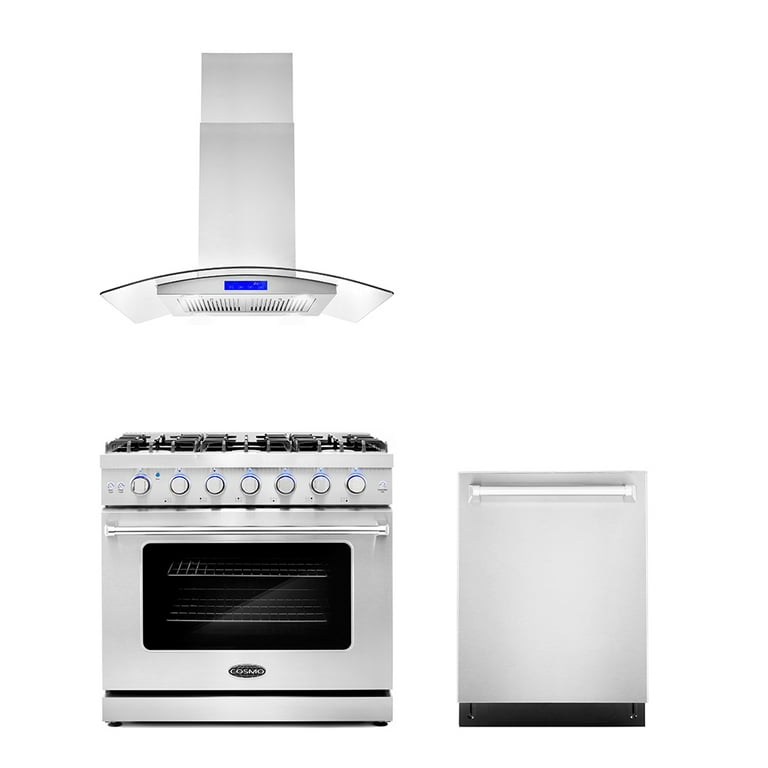The image showcases a collection of sleek, modern kitchen appliances set against a pristine white background. Dominating the scene is a grand, stainless steel gas range positioned on the left. The range features a sophisticated array of seven knobs across its front, hinting at numerous cooking settings. The top of the range reveals a series of gas burners, while its central window allows a peek into the oven's interior, showing two layers of racks. Below the oven is a practical pull-out drawer for additional storage. Above the range, a futuristic semi-circular range hood descends from the ceiling, characterized by clean lines and a glass rectangle at the center housing the controls, with the vent visibly situated underneath. To the right of the range, a smaller, yet equally modern matte silver dishwasher stands out with a minimalist design and a bar handle for easy access, featuring a black bottom accent for a touch of contrast. The overall design is minimalist and contemporary, emphasizing functionality with clean, sleek lines.